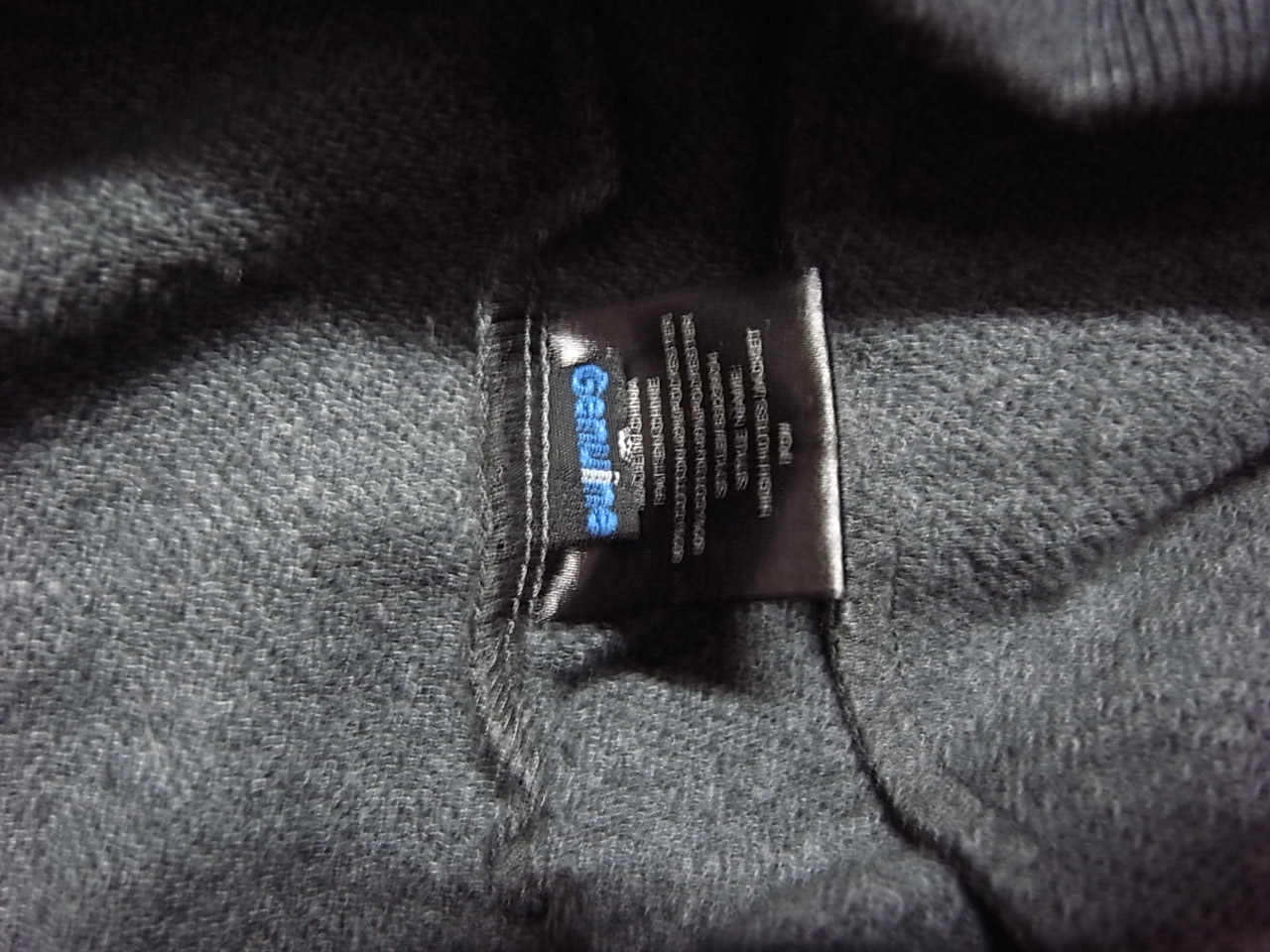A close-up image of a shirt made of finely woven fabric in shades of black and gray, with a particular focus on the textural details. The shirt's material is a soft and subtly lit combination of dark hues, giving it a sleek and elegant appearance. A tag attached to the shirt prominently displays the word "Genuine" in bold white letters, with each letter clearly legible against the dark fabric. The left side of the image is dominated by a deep shadow, which contrasts sharply with the illuminated portions of the shirt, creating a striking visual effect. The tag itself casts a noticeable shadow on the fabric, further enhancing the depth and dimension in the image.